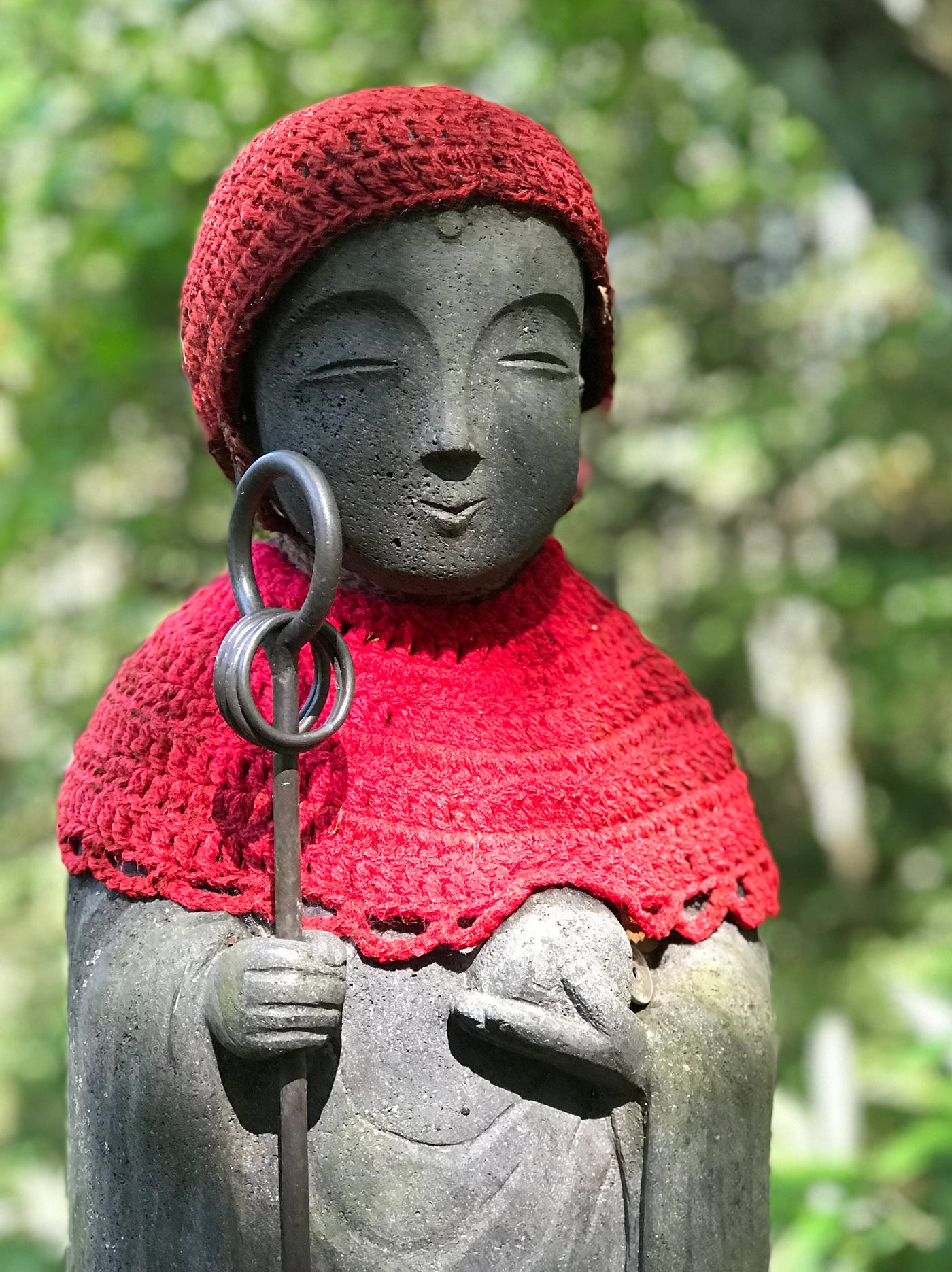In this photo, you are looking at a medium gray stone statue featuring a striking blend of humanoid and artistic elements. The statue is characterized by its expressive face with closed eyes, neatly defined eyebrows, a tiny nose, and a gentle smile. Adorning its head, the statue wears a vivid red knit hat, and around its neck, there is a matching red collar or shawl that extends down to its chest. 

The statue is depicted from the waist up and holds a metal pole in its right hand. This pole is distinguished by multiple rings encircling it near the base and a larger ring at the top. Additionally, the statue’s left arm is positioned in front of its body, with its left hand raised slightly. 

The backdrop of the image is a blurry green scene, suggesting an outdoor environment, likely a forest or garden. The presence of a tree branch in the top right corner enhances this natural setting. The colors in the image prominently include the red of the knit garments, the gray of the stone statue, and the green of the plants in the background, indicating it was taken during the daytime with an emphasis on the statue as the central focus.